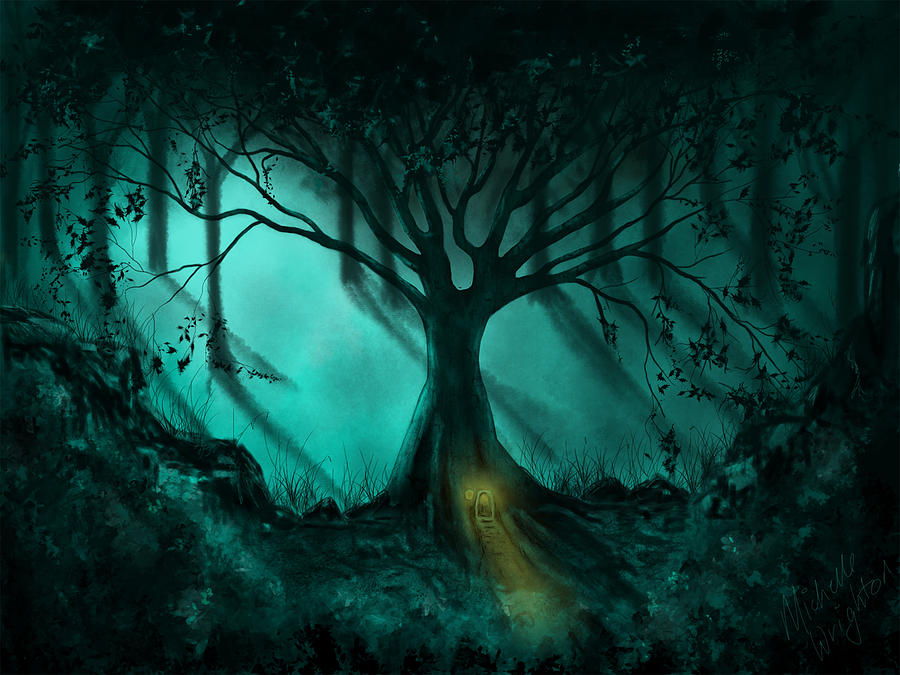The illustration depicts a whimsical, forest scene, reminiscent of artwork seen in children's books. At the center stands a towering, majestic tree with a labyrinth of large branches stretching outward, adorned with a sparse sprinkle of leaves at their tips, some drooping down. Dominating the base of the tree is a tiny, lit-up doorway featuring a softly rounded top, gently illuminating its surroundings as if hinting at a cozy home within the tree. A nearby window and a lamp enhance this enchanted, homely allure. Surrounding the base are patches of dirt, grass, and flowers, contributing to the scene's natural ambience. The forest background reveals shadowed trunks of other tall trees, adding depth and a sense of mystery. The color palette predominantly spans a spectrum of teal, gray, and black, with the vibrant yellow glow from the doorway contrasting sharply against the darker hues. This subtle yet detailed blend of elements conjures an imaginative and serene atmosphere, as if inviting the viewer to step into a fairytale forest.